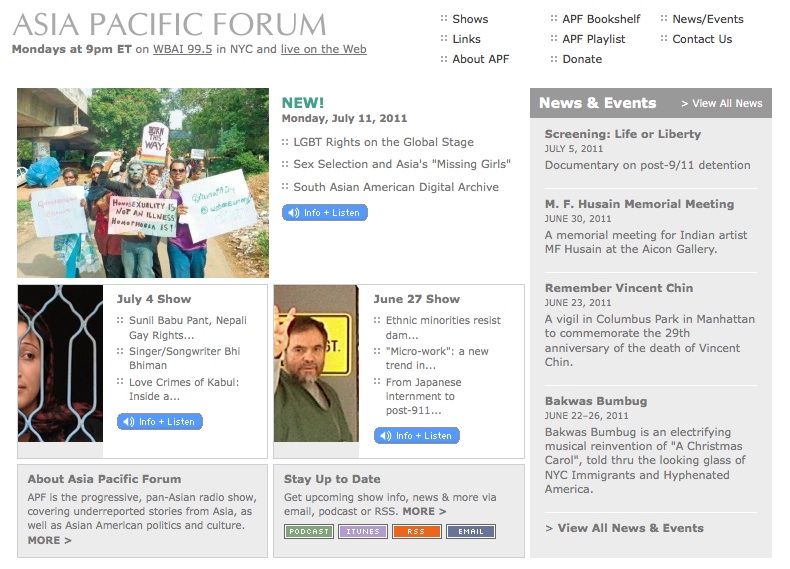This screenshot captures the homepage of the Asia Pacific Forum, prominently displaying its title in the upper left-hand corner. Below the title, it announces that new episodes air on Mondays at 9 p.m. Eastern Time on WBAI 99.5 in NYC, with live broadcasts available on the web. Direct links to the radio station's live stream are embedded in the text.

To the right of this header, there are navigation links arranged in three rows. The first row includes "Shows," "APF Bookshelf," and "News/Events." The second row contains "Links," "APF Playlist," and "Contact Us." The last row features "About APF" and "Donate."

On the left-hand side, the main section exhibits a mixture of text and images. The featured image depicts a protest with signs that read, "Born This Way," "Homosexuality is not an illness," and "Homophobia is." Accompanying this image is information about the new episode airing on Monday, July 11, 2011, which covers topics such as LGBT rights on the global stage, sex selection and Asia's missing girls, and the South Asian American Digital Archive. A blue button labeled "Info and Listen," along with a sound icon, provides access to the episode.

To the right, a gray sidebar titled "News and Events" presents a link to view all news articles. Highlighted events include "Life for Liberty" on July 5, 2011, "M.A. Hussain Memorial Meeting" from June 30, 2011, "Remember Vincent Chin" from June 23, 2011, and "Bakwas Bumbug" running from June 22 to June 26, 2011.

Below this, there is a section with recent show information, detailing the July 4th show, the June 27th show, and an overview of the Asia-Pacific Forum. The description underscores that APF is a progressive pan-Asian radio show focusing on under-reported stories from Asia, as well as Asian American politics and culture.

In the bottom-right corner, options for staying up-to-date are presented with links to podcasts, iTunes, RSS feeds, and email subscriptions.